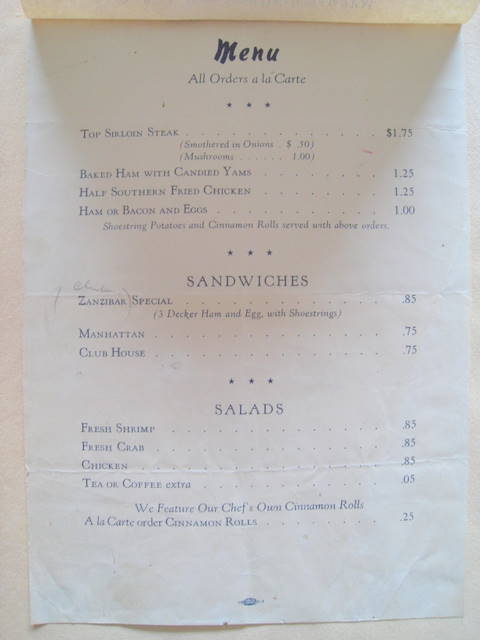A nostalgic vintage menu, printed on white crinkly paper with bold black "Menu" lettering at the top and smaller black print for the details. There is no restaurant name mentioned. The menu offers a variety of à la carte items with remarkably low prices, suggesting it dates back several decades. Entrées include Top Sirloin Steak for $1.75, Baked Ham with candied yams for $1.25, and Half Southern Fried Chicken also for $1.25. Breakfast options feature Ham or Bacon and Eggs priced at $1.00.

The sandwich section lists a "Special" at $0.85, another option illegible but priced at $0.75, and a Club House sandwich for $0.75. Under salads, it mentions Shrimp Salad for $0.85 and Frozen Crab for $0.85, with Chicken Salad also at $0.85. Additionally, Tea or Coffee is available for $0.05. Highlighting the menu, it proudly features the chef's own Cinnamon Rolls, offered à la carte for just $0.25.